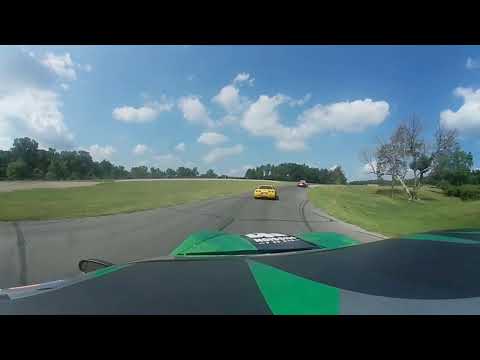The image captures a serene, amateur racetrack on a bright, blue day dotted with puffy white clouds. The photo is taken from inside a sporty black, grey, and green race car, showcasing sponsor logos on its hood. Looking through the windshield, the track curves slightly ahead, with burnout and darker lines visible but no spectator stands or road markings in sight. About 30 feet ahead, a yellow race car leads the way, followed by another red car even further in the distance. The racetrack is flanked by vibrant green grass, clumps of trees, and shrubs, creating a low-key, practice-oriented environment devoid of people or extra text.